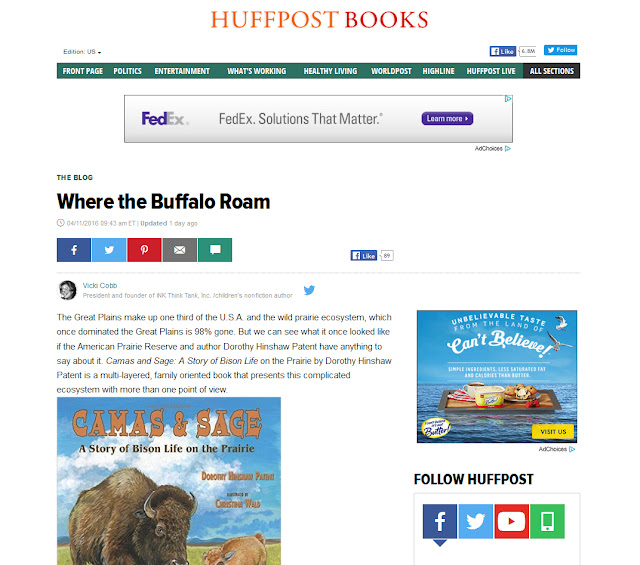Homepage of HuffPost Books

The homepage of HuffPost Books greets visitors with its vibrant orange and red logo displayed prominently. Positioned underneath, the website offers several navigation options, including an "Edition" dropdown initially set to "US". Social media interaction buttons are also present, such as a Facebook "Like" button and a blue "Follow" button for Twitter.

The website’s sections are clearly categorized, offering quick access to various topics including Front Page, Politics, Entertainment, What's Working, Healthy Living, World Post, Highline, HuffPost Live, and a comprehensive "All Sections" option for further exploration.

A notable FedEx banner ad is featured, promoting "FedEx Solutions That Matter" with a purple "Learn More" button inviting users to discover more.

Highlighted on the homepage is a blog piece titled "Where the Buffalo Roam," dated April 11, 2016, authored by Vicky Cobb, the president and founder of the NK Think Tank. Cobb discusses the Great Plains, which constitute one-third of the USA, and the diminishing wild prairie ecosystem, now 98% gone. The blog draws attention to efforts by the American Prairie Reserve and author Dorothy Hinshaw Patent to preserve and illustrate what the landscape used to be.

A featured book image accompanies the blog, showcasing "Kamsin Sage: A Story of Bison Life on the Prairie" by Dorothy Hinshaw Patent. The cover displays large bison grazing in a grassy field under a clear blue sky. The book is described as a multi-layered, family-oriented narrative, providing varied perspectives on the intricate prairie ecosystem.